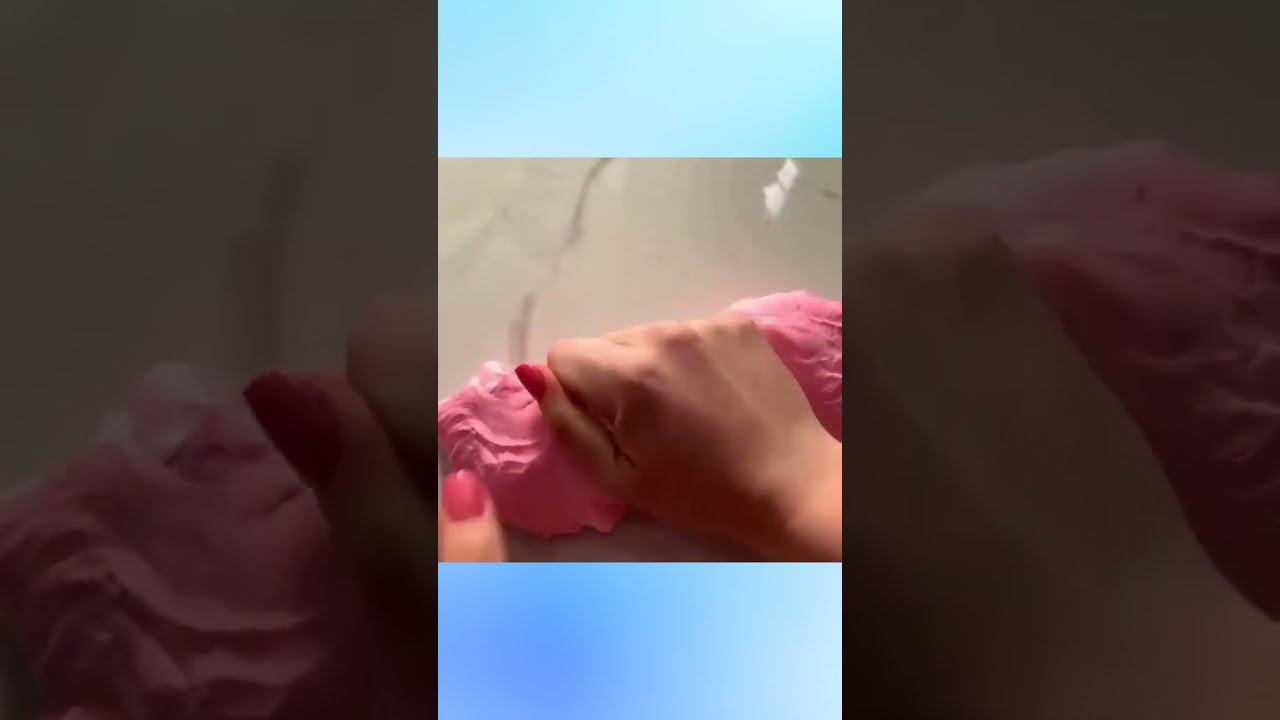In this photograph, a centrally focused image displays a right hand with pink nail polish on the left thumb, kneading or shaping a lump of pink dough or clay. The primary background is light gray, possibly a shiny marble countertop. This central image is framed horizontally above and below by medium blue bars on a white background, giving the whole scene a landscape orientation while the main image remains portrait-oriented. The left and right sides of the image feature black rectangles showcasing blown-up, darkened details of the same hand and pink material, further enhancing the central theme in a mirrored and magnified manner.